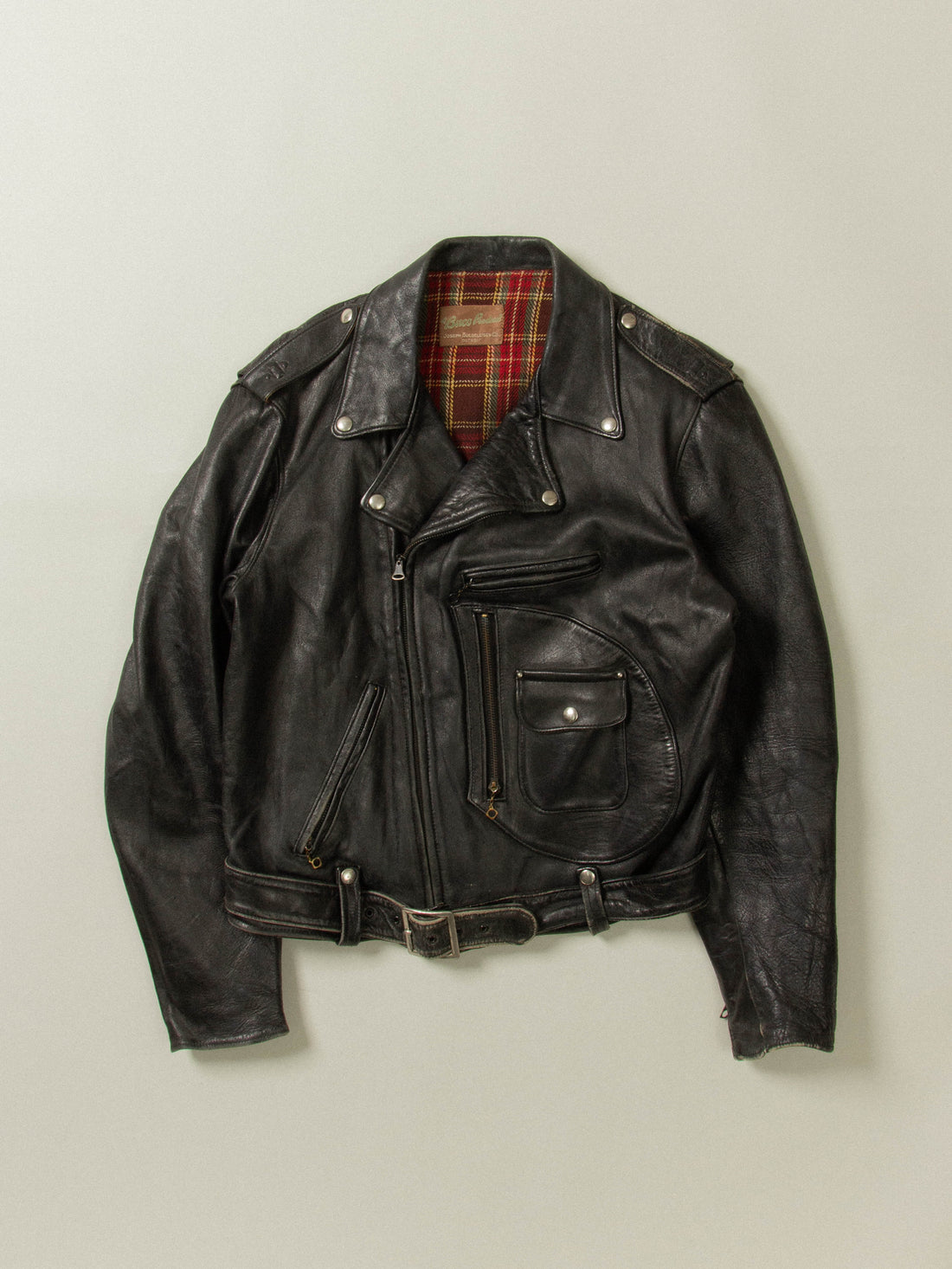The image showcases a black leather jacket, possibly from the 1950s, displayed mounted on a wall. The jacket, though worn frequently, retains a soft texture and features a red and possibly gold and green plaid lining inside. It is waist-length and sports an array of hardware details, which include epaulets with metal snaps on the shoulders and additional metal snaps at the corners of the collar. The front of the jacket features an off-center zipper slightly to the left, complemented by a belted waist that allows further closure. Several pockets enhance its functionality: a diagonal pocket on the left, a large vertical round pocket with a smaller zippered pocket on top on the right, as well as a chest pocket above it. Each sleeve ends with a zipper. A tan leather label with unreadable writing is also visible inside the collar. The jacket is displayed against a light-colored, likely white, surface.